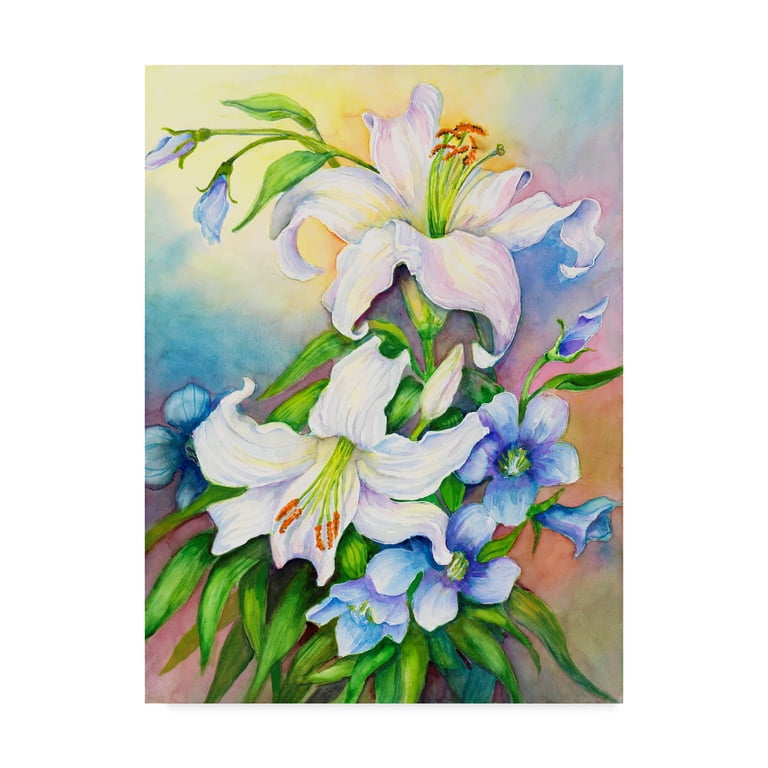This is a detailed painting of a bouquet of flowers set against a vibrant, pastel-like background blending shades of blue, yellow, purple, and orange. Dominating the bouquet are two large white flowers with big, droopy, and somewhat wiggly petals. The central white flower has six distinct petals and long, green filaments with red-tipped ends emerging from its center. Nearby, another large white flower points to the bottom left, featuring similar green filaments with frizzy red tips. 

Complementing the white flowers are several blue flowers, varying in position and development. The right side of the composition showcases a cluster of light blue flowers, each having five to six petals that transition to white or lighter blue at the edges. These flowers appear stacked, with some fully open and others still closed and undeveloped. Additional blue flower buds, similarly light blue but still in bud form, are positioned at the top left.

Surrounding the flowers are numerous green leaves, enhancing the natural bouquet aesthetic. The backdrop, a mix of pastel hues resembling a gently blended rainbow, adds depth and a dreamy quality to the painting, suggesting an outdoor setting during the day. The colors range from pale yellows in the top left to blues, pinks, oranges, and darker grays toward the bottom right, creating a harmonious and colorful canvas.